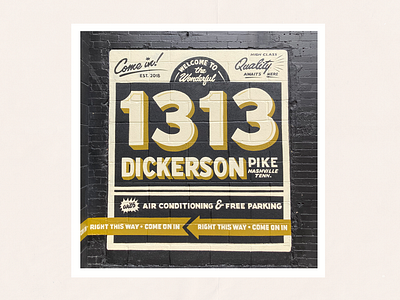This image depicts a vintage-style advertisement on a black brick wall, painted to create a nostalgic feel. The ad is primarily on a tan or light pink background, framed by a white border, with a central black rectangular bar. At the top, there's a black half-circle bearing the inscription "Welcome to the Wonderful" in black lettering. To the left in cursive, it reads "come in," and to the right, "Quality," with smaller illegible text beneath it. A larger black border in print features the address "1313 Dickerson Pike, Nashville, Tennessee." Below this, another black bar highlights amenities with the text "Air Conditioning and Free Parking." Beneath this section, there are orange-yellow arrows with white text pointing leftwards, stating "right this way, come on in, right this way, come on in." The ad appears glossy under light, suggesting it might be an art print or a polished sign.